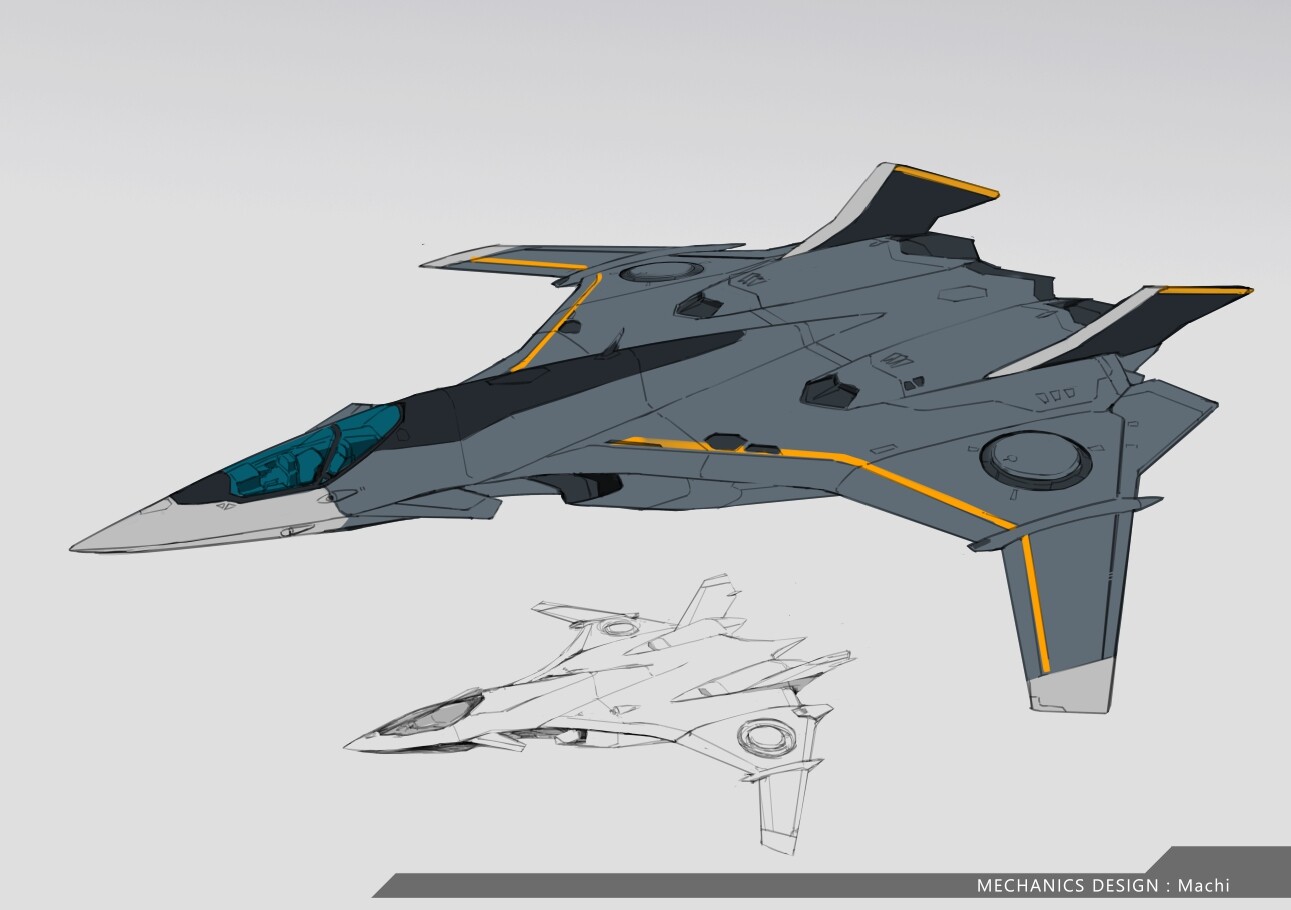The image features a detailed and futuristic-looking drawing of a jet or spacecraft, primarily gray with striking yellow stripes running along its wings. The sleek and thin design of the jet is accentuated by a long fuselage and a pointed nose, rendered in light gray. The cockpit is highlighted by a blue-tinted windshield, adding a modern touch. The wings jut out to the sides, ending in black spoilers, and two symmetrical circular designs adorn each wing. Beneath this colored drawing, there's an identical, smaller sketch done entirely in black lines, devoid of the yellow, gray, and blue hues of the upper image. The jet appears to be in flight, but with no visible pilot inside the cockpit. The simplistic light gray background features a horizontal strip at the bottom with white text reading "Mechanics Design: MACHI." This cool, airborne design is likely a conceptual or prototype drawing of an advanced jet.